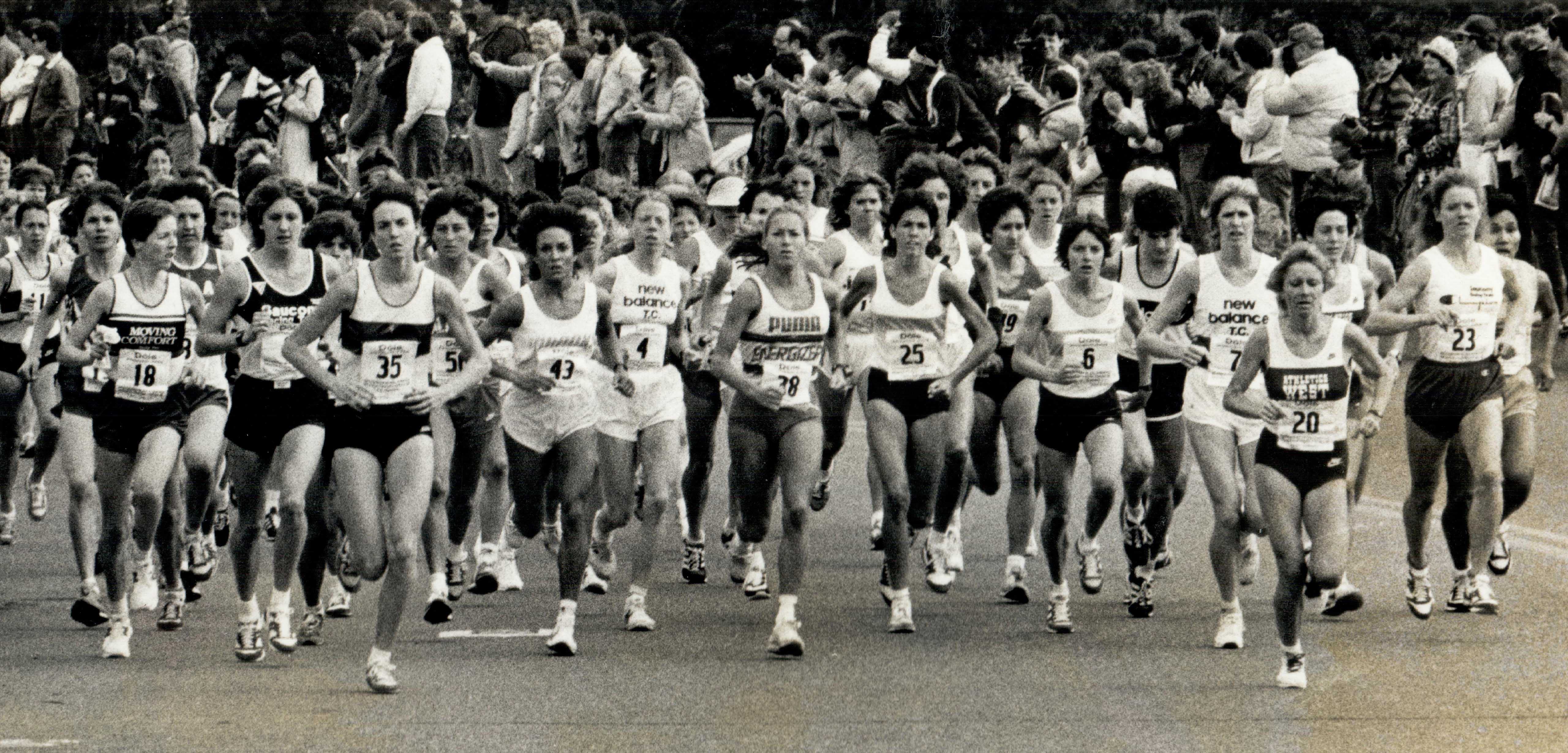This is a black-and-white photo likely from the 1970s or 1980s capturing a marathon scene. The composition is a wide-angle shot with the camera placed in the middle of the street facing the oncoming runners. Approximately 30 athletes, primarily women, are running toward the camera, dressed mostly in tank tops and running shorts with bib numbers such as 25, 43, and 18. Some of the shirts feature various brand names like New Balance and Puma Energizer, though the text is not easily readable. The background reveals a crowd of spectators, a mix of men and women of various ages, who are mostly looking to the left rather than at the runners. Some crowd members appear to be holding cameras. The bottom of the image shows the gray pavement, adding to the authenticity of the scene.